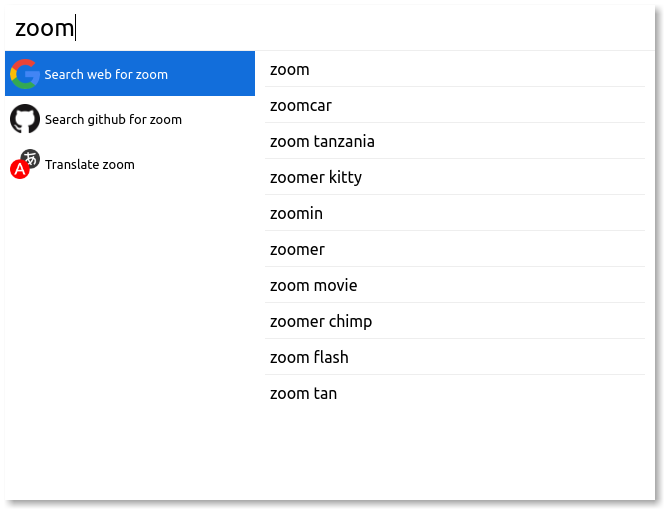The image showcases a user interface display, likely from a web browser or an application, demonstrating a search results screen for the term "Zoom." The background is predominantly white, providing a clean and simple backdrop for the content.

In the upper left corner of the screen, there is a white search bar with the term "Z-O-O-M" typed into it. Directly below this search bar is the primary section titled "Search Web for Zoom," which is highlighted in blue with white text, indicating it is the active selection. 

To the right of this section, there's a vertical list of related search suggestions in black text. The suggestions include: 
- Zoom
- Zoom Car
- Zoom Tanzania
- Zoomer Kitty
- Zoom In
- Zoomer
- Zoom Movie
- Zoomer Chimp
- Zoomer Flash
- Zoomer Tan

Below the "Search Web for Zoom" section, two additional options are presented. The first is "Search GitHub for Zoom," which appears to feature a GitHub icon resembling a cat within a circle. The second option is "Translate Zoom," displaying an icon with the letter 'A' and a corresponding Japanese character, symbolizing translation capabilities.

Overall, the image seems to illustrate the process of conducting a web search for the term "Zoom" and highlights various interface elements and related functionalities within the page.